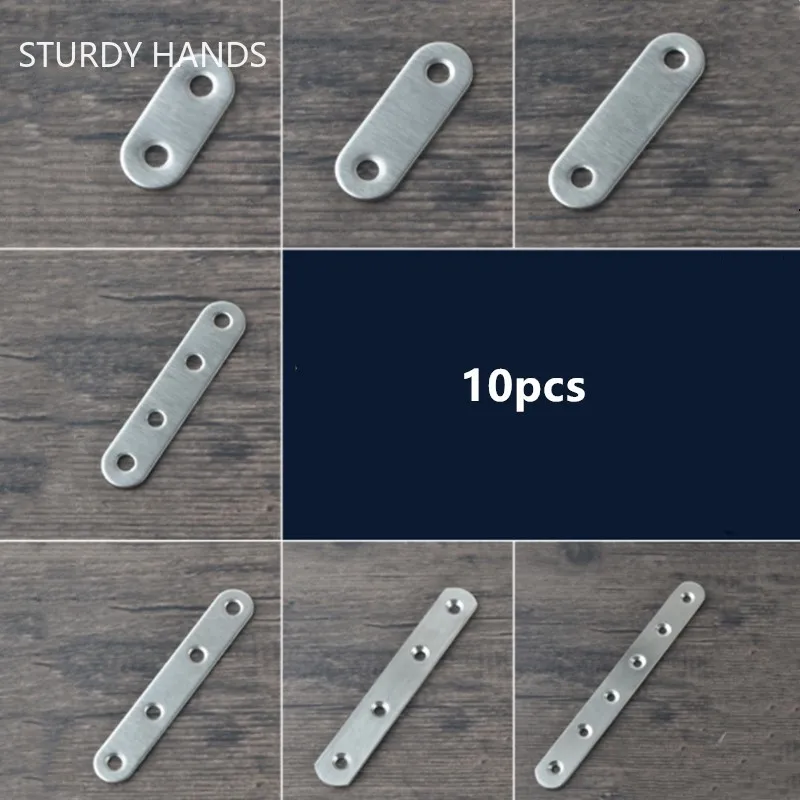This is an image of a poster featuring various metal plates used for handiwork. The top left corner displays the text "Sturdy Hands," likely indicating the brand. The center of the poster contains a black box with the phrase "10 PCS" signifying the contents of the set. Arranged in a 3x3 grid, seven sections showcase long, oval-like metal pieces of varying lengths, positioned on a dark wooden or faux wooden background that resembles a table. Each piece features different configurations of punch holes: some have two holes, others have four, and one elongated piece has six holes. The pieces vary in length and hole arrangement, displaying a practical range of options for securing materials with screws. The visual emphasis and detailing suggest the product's versatility and durability for various DIY or professional projects.